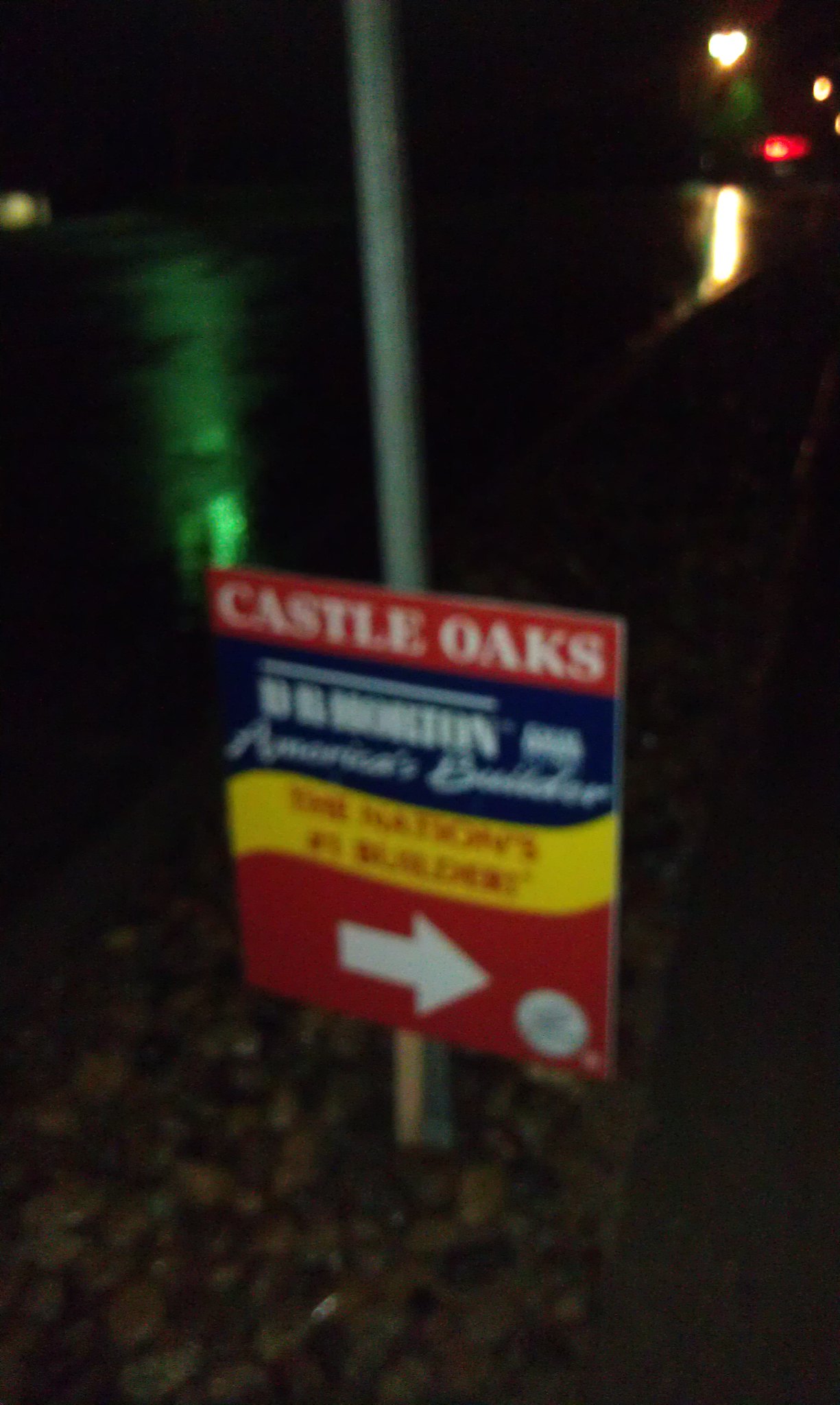In this night-time outdoor digital photo, the background is predominantly dark, showcasing a night sky in the uppermost part. The image centers on a slender, slightly tilted gray metal pole, mounted almost at the middle of the photo. This pole supports a square-shaped sign positioned low on it. The top part of the sign is red with the white text "Castle Oaks." Below, there is an unreadable blue strip, followed by a yellow section with blurred red text. The bottom of the sign is also red, featuring a white right-pointing arrow and a small white circle in the lower right corner.

In the background, on the right side, two street lamps emit yellowish light, creating reflections on what seems to be recently paved and wet asphalt. These reflections form long streaks, with visible puddles particularly on the left side of the image. There are additional reflections of yellow and green lights on the road. Low green shrubbery appears near the bottom of the image, highlighting the outdoor setting of this photograph.